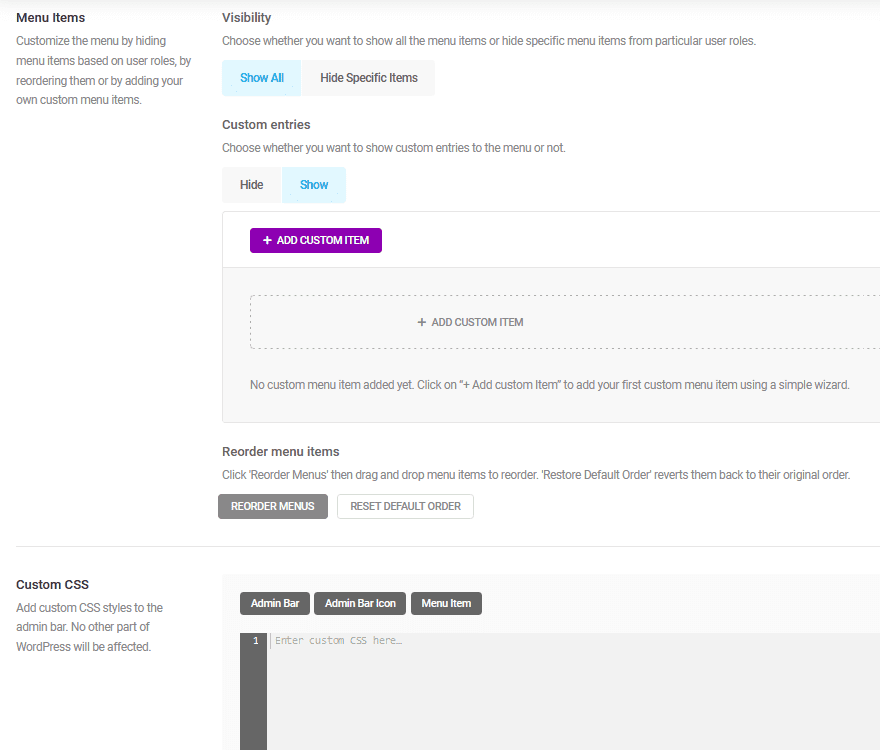This image depicts a user interface screen for customizing a menu based on user roles and adding custom entries. On the side tabs, there are various menu items that users can adjust. 

- **Menu Customization:** 
  - Users can hide menu items from specific user roles.
  - Reorder existing menu items.
  - Add new custom menu items.

- **Visibility Settings:** 
  - Options to show all menu items.
  - Alternatively, hide specific items based on user roles.

- **Custom Entries:**
  - Option to display custom entries in the menu.
  - An 'Add Customs' bar where users can add custom menu items using a wizard.
  - Display message indicating "No custom menu item added yet."
  - Instructions prompt: "Click on add items to add your custom menu item using a simple wizard."

- **Menu Reordering:**
  - A section at the bottom provides options to reorder menu items by dragging and dropping.
  - Includes a 'Restore Default Order' button to revert the menu to its original configuration.
  - Buttons labeled 'Reorder Menu' and 'Reset Default Order.'

Additionally, on another tab at the bottom, there is an option to "Add custom CSS styles to the admin bar."

The layout is organized and user-friendly, guiding users through the process of menu customization and management with clear instructions and interactive elements.